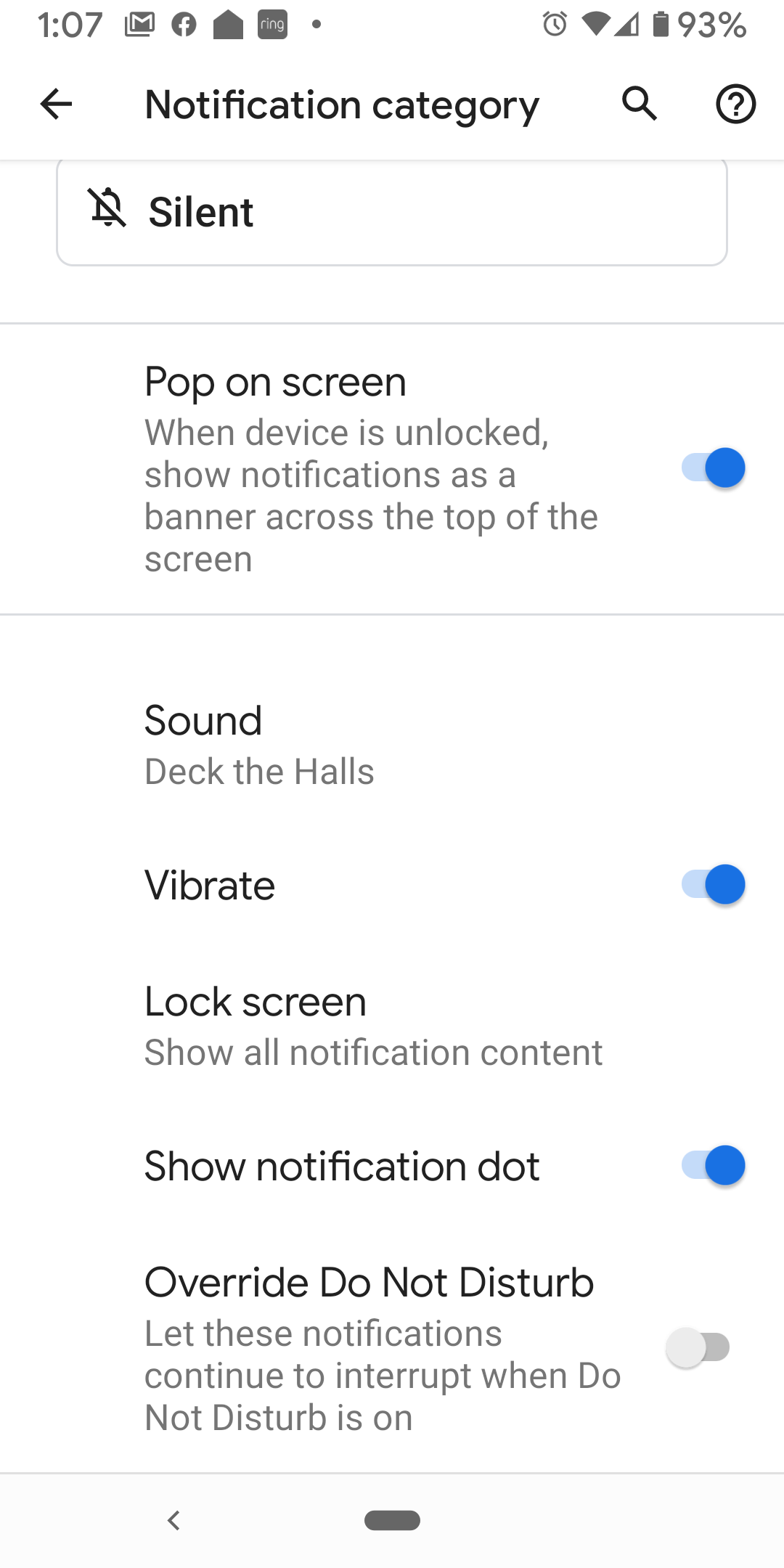The screenshot presents a smartphone settings interface with a black background and white foreground. The status bar at the top displays the current time, background icons, and signal strength. Below, the main screen focuses on Notification Category settings.

A navigation arrow on the left suggests the option to return to the previous menu. The first listed setting is "Silent," indicated by a bell icon with a slash through it, confirming that silent mode is currently activated. 

Following this is the "Pop Up on Screen" setting, configured to display notifications as banners across the top when the device is unlocked; this setting is enabled.

The next setting pertains to sound notifications, specifically set to "Deck the Halls." This is followed by the "Vibrate" setting, which is toggled on.

For the "Lock Screen," notifications are set to show all content, although there is no corresponding toggle button visible for this option. The "Show Notification Dot" setting is enabled, allowing for notification indicators on app icons. Lastly, the "Override Do Not Disturb" option, which would allow notifications to bypass the Do Not Disturb mode, is turned off.